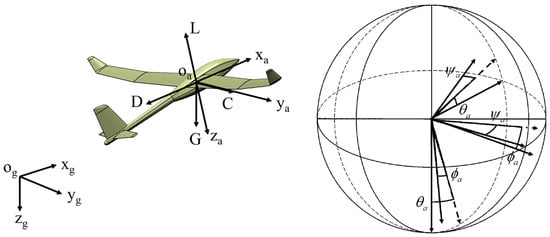The image is a detailed technical diagram set against a plain white background, measuring roughly four inches wide by two inches high. In the lower left corner, three arrows converge at a point labeled "Og" (with a small 'g' subscript). Each arrow represents an axis and is labeled as follows: Zg points downward, Yg points horizontally to the right, and Xg points diagonally upward to the right.

Centered above and to the right of these arrows is an illustration of a light greenish-gray model plane. The plane has a cylindrical body and slightly curved wingtips. A set of crisscrossing black arrows is superimposed on the plane, indicating various forces and directions. These arrows are labeled L (upward), D (angled downward to the left), G (downward), C (diagonally downwards to the right), Xa (right and slightly upward), Ya (downward and right), and Za (downward). The central point where these arrows intersect is marked "Oa."

To the far right of the image, there is a diagram of a sphere with a network of lines and arrows depicting radii and mathematical symbols, including Greek letters. The sphere is traversed by horizontal and vertical lines resembling latitude and longitude, giving it a globe-like appearance. Various radii labeled with equations, such as "Qa" and "Oa," extend from its center towards the upper right quadrant.